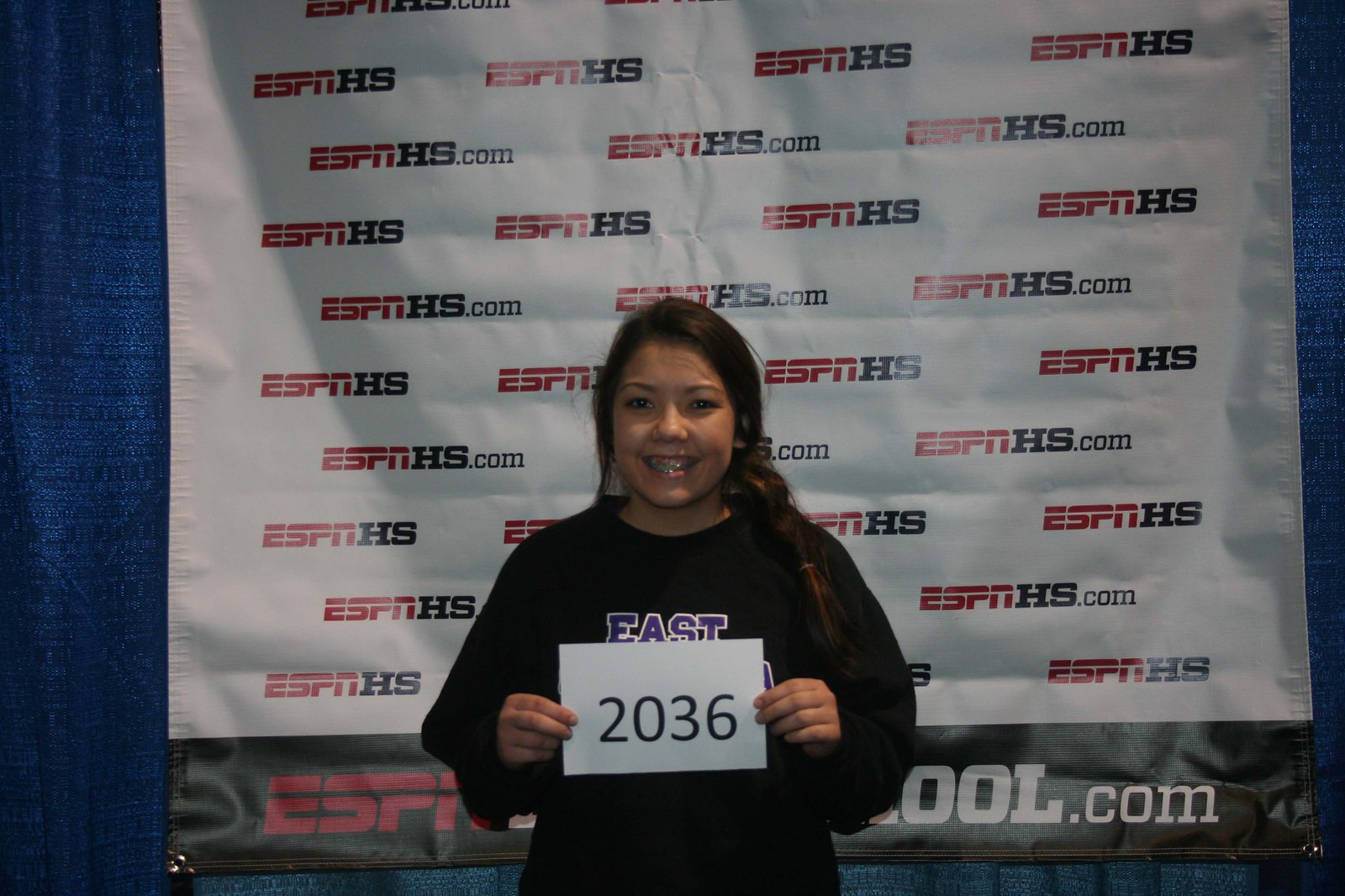This horizontally aligned rectangular image features a young woman smiling at the camera, with braces visible on her teeth. Her long brown hair is styled in a braided ponytail draped over her left shoulder. She is holding a rectangular sheet of white paper horizontally, displaying black numbers reading "2036." She is dressed in a black sweatshirt adorned with a purple print of the word "East," partially obscured by the paper she is holding. 

In the background, there is a large banner with a white upper section and a black lower section, prominently featuring the logo "ESPNHS" in a repeating pattern. The "ESPN" is printed in red while "HS.com" is in black. This pattern continues across the banner, and a larger "ESPN" logo is visible at the bottom, partially covered by the girl, with "OOL.com" discernible on the right side. A tall blue curtain or wall is behind the banner, visible on the sides of the image.

The overall scene suggests that she is at some form of award or recognition event possibly organized by ESPN or related to ESPNHS.